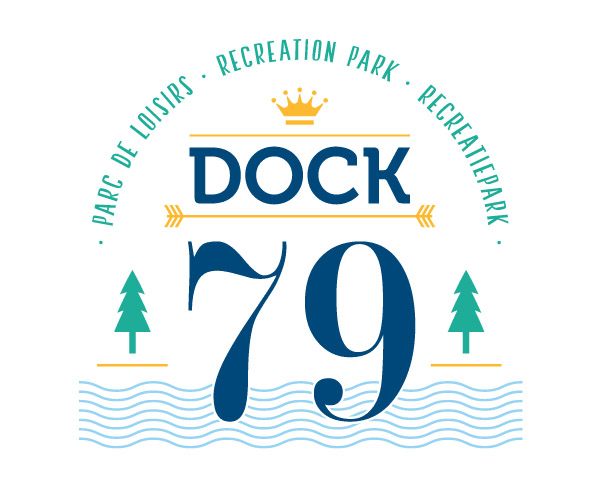The image is a logo on a white background, depicting a recreation park. At the center is the highly stylized number "79" in bright blue, with wavy blue lines below it representing water. On either side of the "79" are stylized blue trees, each with a short gold line below them. Above the "79" is a gold line with angled ends, resembling a bi-directional arrow with flights on both sides. Positioned above this line is the word "DOCK" in bright blue letters, framed by two yellow lines—one above and one below. Topping the logo is a yellow crown with the phrase "Recreation Park" arched above in blue text, expressed in three different languages, including "park de loisirs."